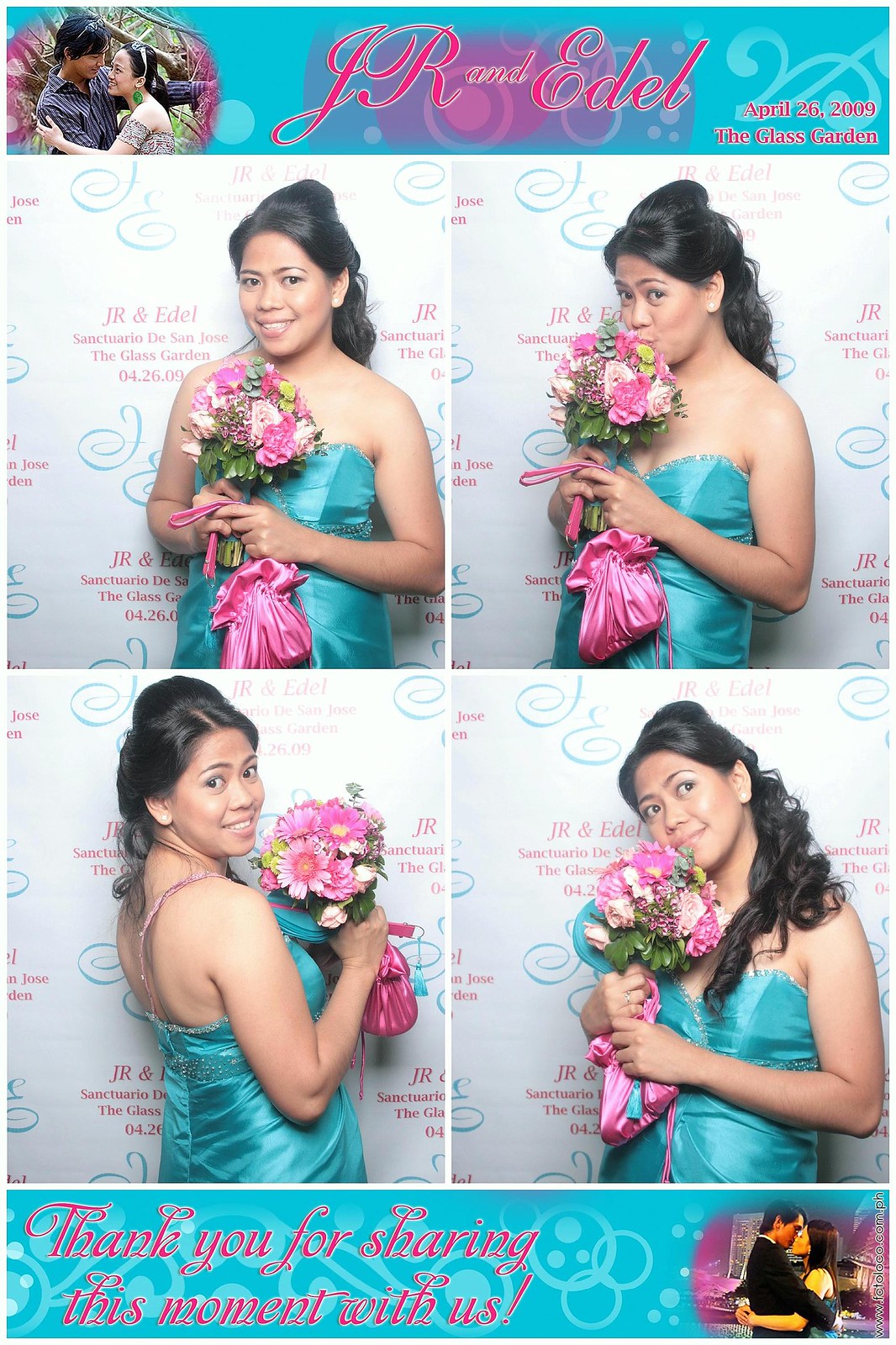In this image, we see a series of four photographs featuring a young woman with black hair tied up behind her head. She is wearing a blue strapless dress and holding a bouquet of pink, white, and yellow flowers, along with a pink silk bag dangling from her hands. In the top left photo, she is standing while holding the bouquet; next to it, she is smelling the bouquet raised to her face. The bottom left photograph shows her with her back turned, holding the bouquet while glancing back at the camera. Lastly, the bottom right photo captures her gazing into the distance with the bouquet close to her face. Above these photos, the text reads: "J.N.R. & Edel, April 26, 2009, The Glass Garden." Below the images, it says: "Thank you for sharing this moment with us." 

Additionally, the image includes a background featuring a couple, presumably J.R. and Edel, embracing and kissing under red text that reads "J.R. & Edel, April 26, 2009, The Glass Garden." The couple appears to be enjoying a special, possibly wedding-related, event.